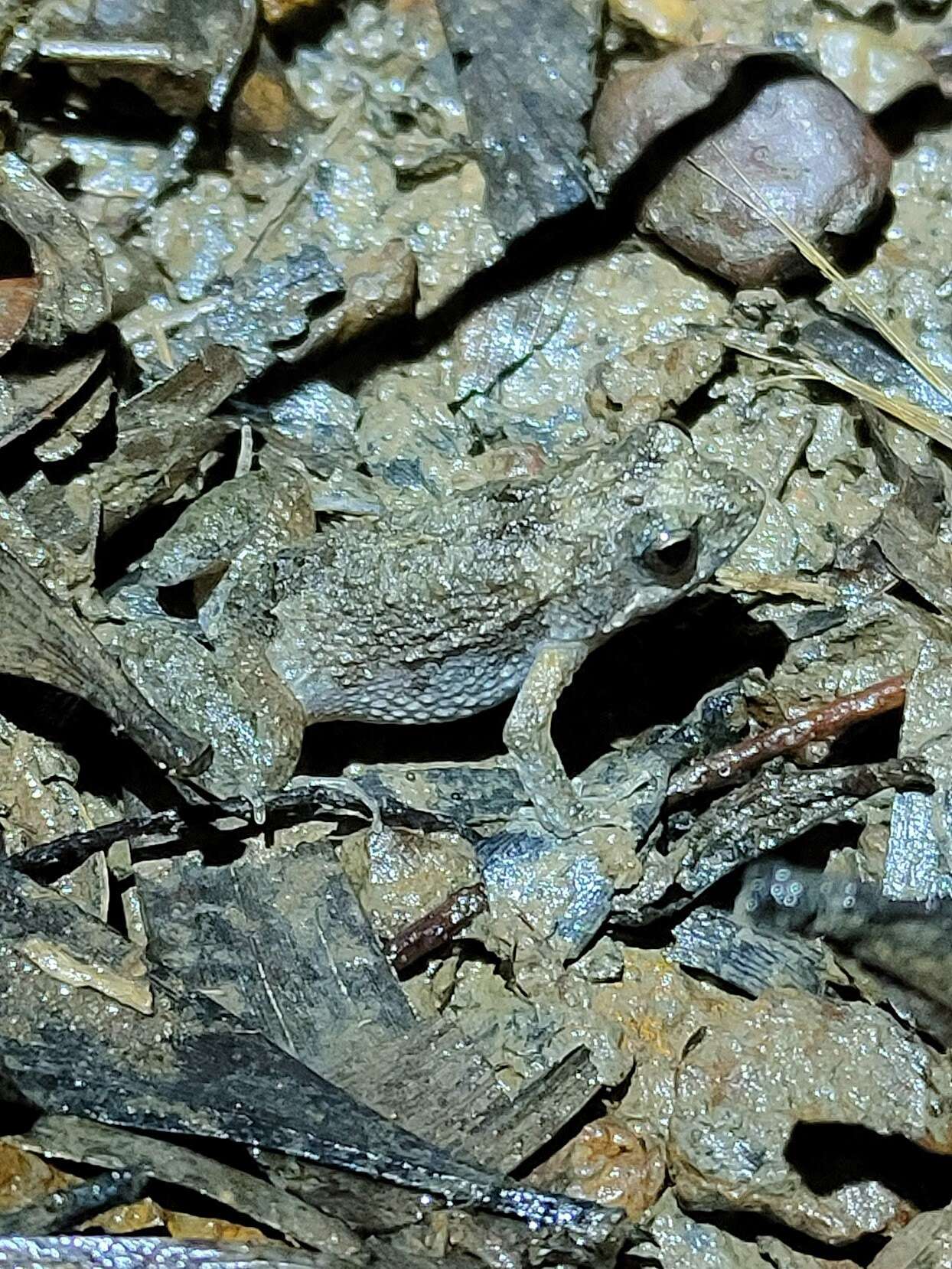In this detailed photographic image taken outdoors during daytime, a small brown toad with subtle gray splotches effortlessly blends into a muddy, rock-strewn environment. The toad, positioned diagonally from the bottom left to the top right at a 30-degree angle, has its right arm visible and faces towards the right side of the image. Its camouflaged skin mirrors the brown rocks adorned with similar gray splotches, making its presence almost undetectable except for its distinctive eyes and tapered mouth. The setting hints at a rainforest floor with wet, shiny rocks, moist leaves, sticks, and possibly dead plants, suggesting recent rainfall and proximity to a water source. Sunlight overhead casts a shadow on the toad and highlights a dry leaf in the upper right corner, adding a touch of contrast to the otherwise damp surroundings.